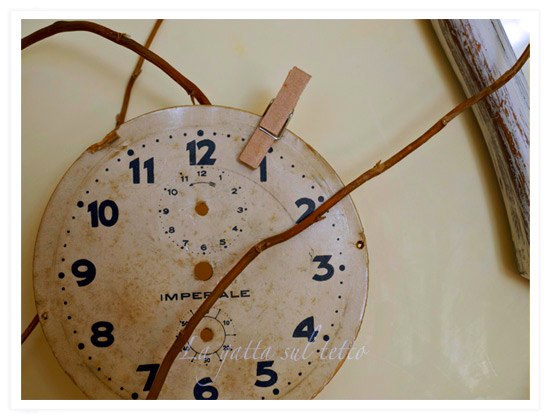The image depicts an old, dirty white clock face showing black numbers 1 through 12 with a smaller clock for seconds below the large 12. It is marked "Imperial" in the center. The clock is against a tan or beige background, perhaps a wall, and appears to be non-functional, as it has no hands and is quite scratched and dingy. Brown wires or sticks seem to be attached to the clock, possibly serving as makeshift supports. In the upper right corner, there is a clothespin attached to the clock face and what appears to be part of a window pane or mirror. Additionally, there are brown sticks crisscrossing behind the clock and a long brown piece of wood positioned diagonally from the lower left to the upper right in the upper right corner. The background and objects give the impression of an artistic, vintage display. On top of the image, in white text, it reads "L-A-G-A-T-T-A-S-U-L-T-E-T-T-O."